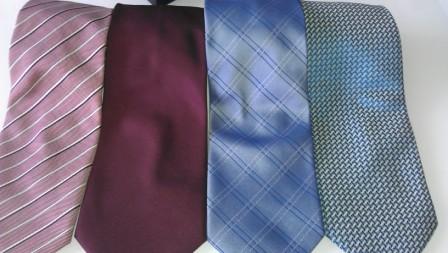The photograph showcases four men's dress ties laid out on a white table, with the top and bottom edges of some ties cropped out. From left to right, the first tie is a salmon pink with black and white diagonal stripes, though its color gives an impression of pinkish light purple with dark purple and white stripes. The second tie is a dark red-burgundy, shimmering in the light and appearing as a solid wine color. The third tie is a light bluish-gray, exhibiting a shiny texture with a dark blue crisscross pattern. Lastly, the fourth tie is a greenish pattern, although it can be perceived as a gray-blue tie with a small, intricate white houndstooth design providing a textured appearance. The ties are arranged in a way that they appear to flow from top to bottom, emphasizing their variety in colors and patterns.